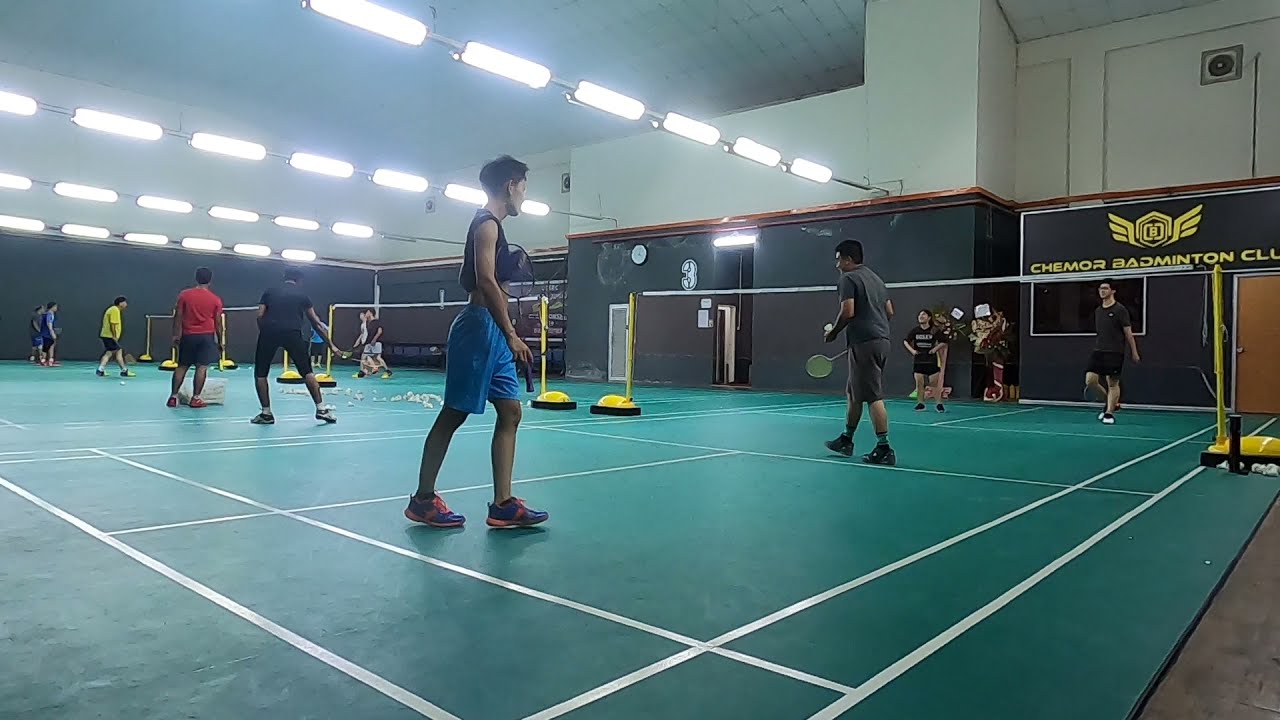The image captures a bustling indoor gym with four visible badminton courts. The courts are lined with white segments on a dark blue-green floor and are equipped with nets held up by yellow poles. Most courts feature two players on each side engaged in a lively match, wielding their rackets. Above the courts, bright fluorescent lights illuminate the scene, while some courts also have strings of glowing white rectangular lights suspended over them. The players, dressed in sleeveless tops or short-sleeve shirts and shorts, are in various stages of play. Spectators can be seen watching from the sidelines. In the background, the lower half of the wall is painted dark gray, transitioning to light gray on the upper half. Notably, on the far right side of the background, a yellow emblem featuring a hexagon with zeros in the center and wings on each side is visible. Below this emblem, partially obscured, the text reads "Keymore Badminton Club," with the letters "U-M-B" in "Club" cut off.